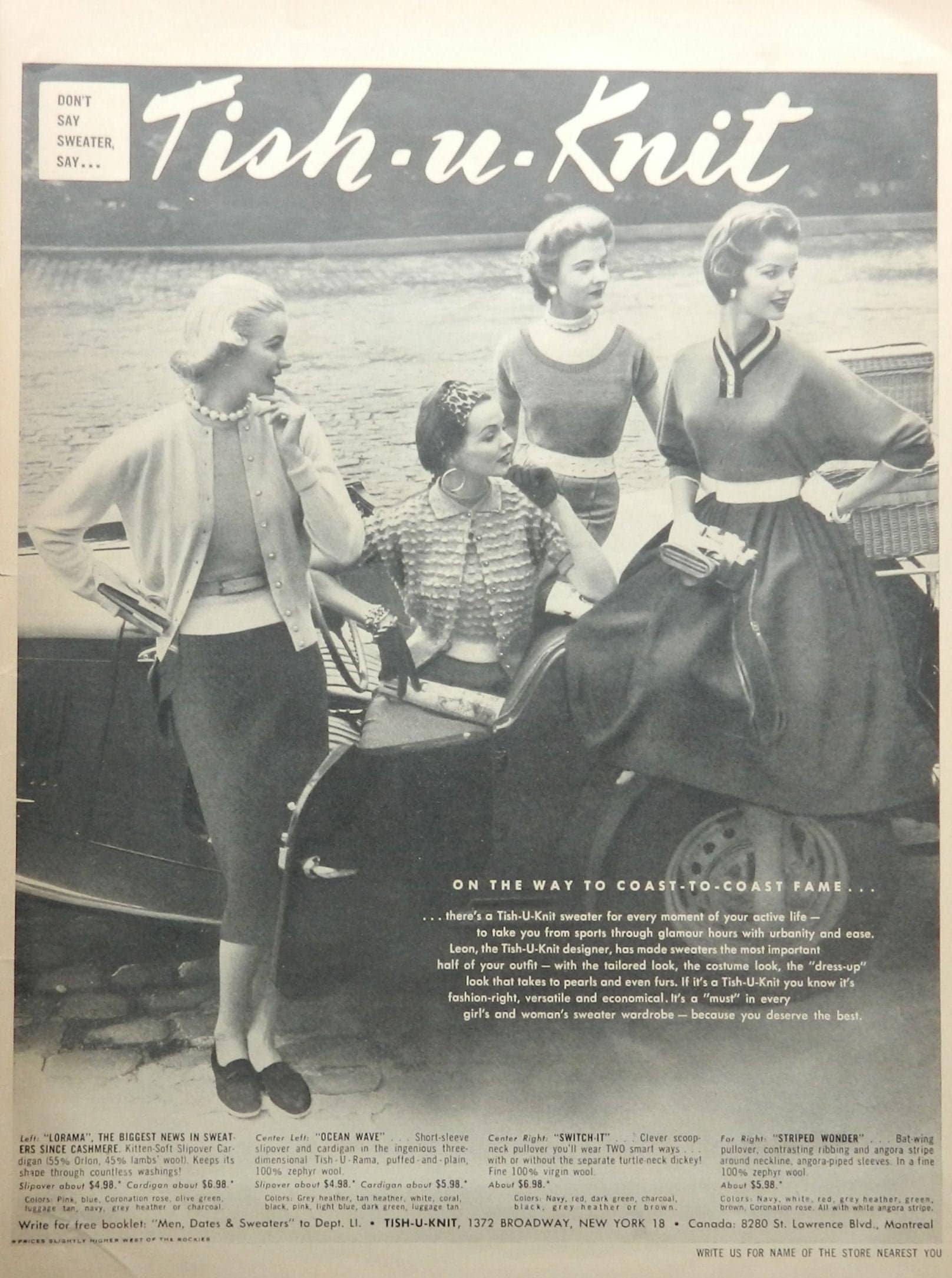This vintage black and white advertisement, possibly from the 1940s, showcases the slogan "Don't say sweater, say Tissue Knit" prominently displayed within a white box at the top left. To its right, bold white font spells "Tissue Knit." The scene is set with four stylish women positioned around a classic convertible sports car, parked by a river, with sandy terrain underfoot. Each woman exudes a chic elegance with their elaborately styled short hair and fashionable attire, comprising knitted sweater tops, cardigans, and dresses.

One woman, adorned with a pearl necklace and sporting short, blond hair, stands on the left. Another, sitting in the car, accessorizes with a hoop earring, black gloves, and a bandana tied around her forehead. The two women to the right of the car both showcase short hairstyles and wear distinct dress styles; one in a striped top and skirt, and the other in a dress belted at the waist. Several models strike dynamic poses with hands on hips or raised to their faces, all gazing toward an unseen point off-camera to the right.

Below this captivating scene, detailed text likely describes the products and their prices, including sweater names such as Striped Wonder, Stitch It, Ocean Wave, and Larama. Further enhancing the authenticity of the ad is the inclusion of a New York address: 1372 Broadway, New York, 18, tying the entire vintage promotional piece together.